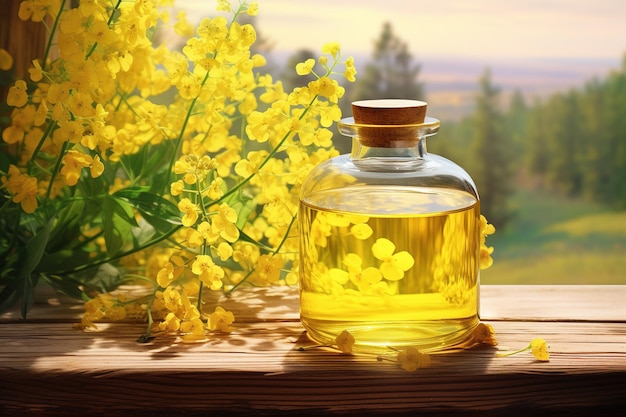In this outdoor scene, the sky forms a backdrop to a picturesque landscape featuring either an ocean or a river with blue water shimmering in the distance. The foreground is dominated by a sturdy wooden windowsill or table adorned with a collection of bright yellow flowers. These flowers, with their green leaves and thin, delicate stems, are vividly open and vibrant, adding a splash of color to the setting. Alongside these flowers is a stout, clear glass bottle, nearly filled with a yellowish liquid, possibly olive oil. The bottle is topped with a brown cork stopper. Surrounding the bottle, some of the yellow flowers and additional leaves are either resting on the surface or positioned behind the bottle. Pine trees, likely evergreens, and patches of green grass fill the background, weaving together layers of natural beauty in this captivating and serene image.